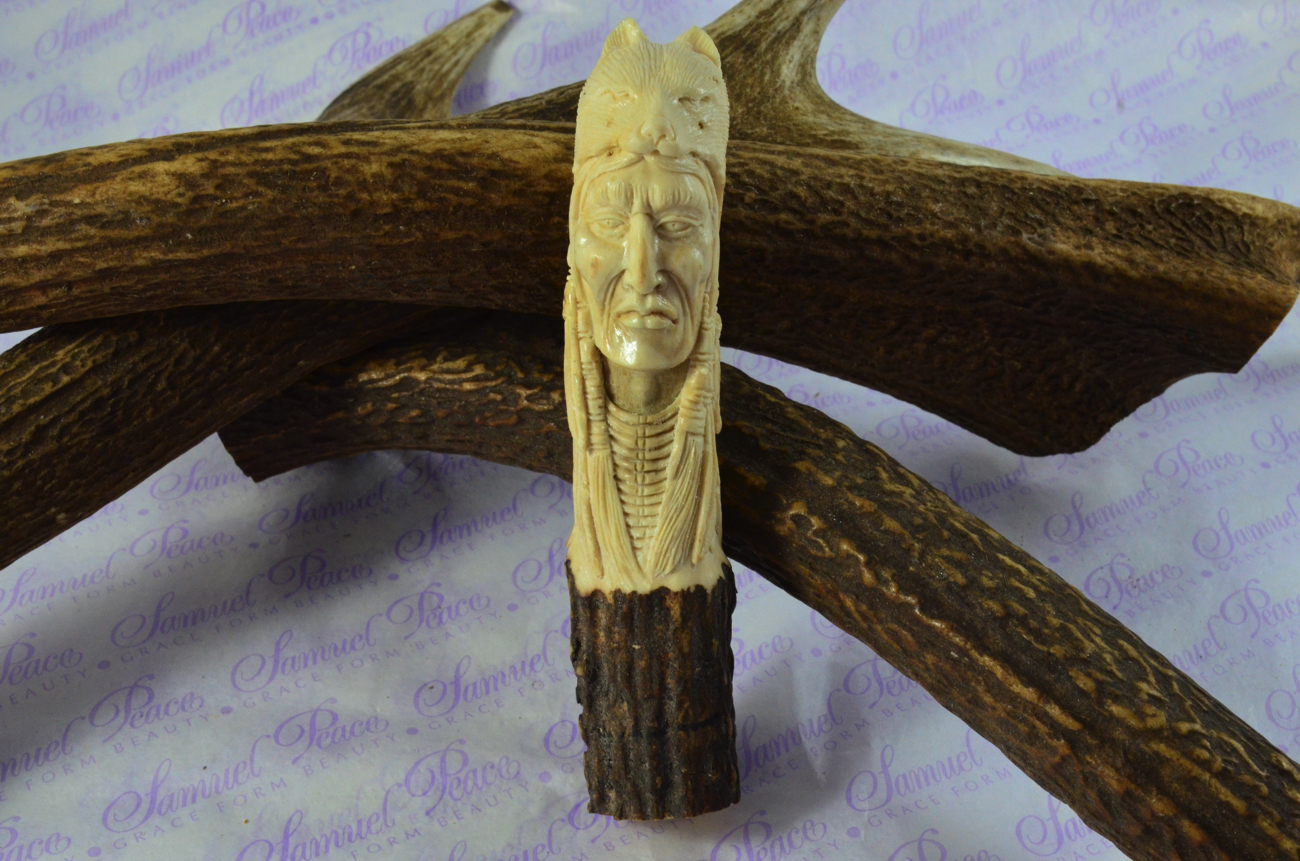The photograph showcases a meticulously detailed carving of a Native American shaman, intricately sculpted from a piece of ivory-colored wood. The shaman is depicted with long braids and a headdress that appears to be adorned with the head of a lion, tiger, or wolf. His pronounced nose adds to the realism of the sculpture. The carving is surrounded by uncarved, brown and gold-colored wooden logs that support and frame it. The whole arrangement is set against a white parchment background repeatedly imprinted with the name "Samuel Peace" in blue or violet lettering. This likely indicates the artist behind the creation. The background parchment and the supportive wood enhance the elegance and focus on the central ivory-colored carving.